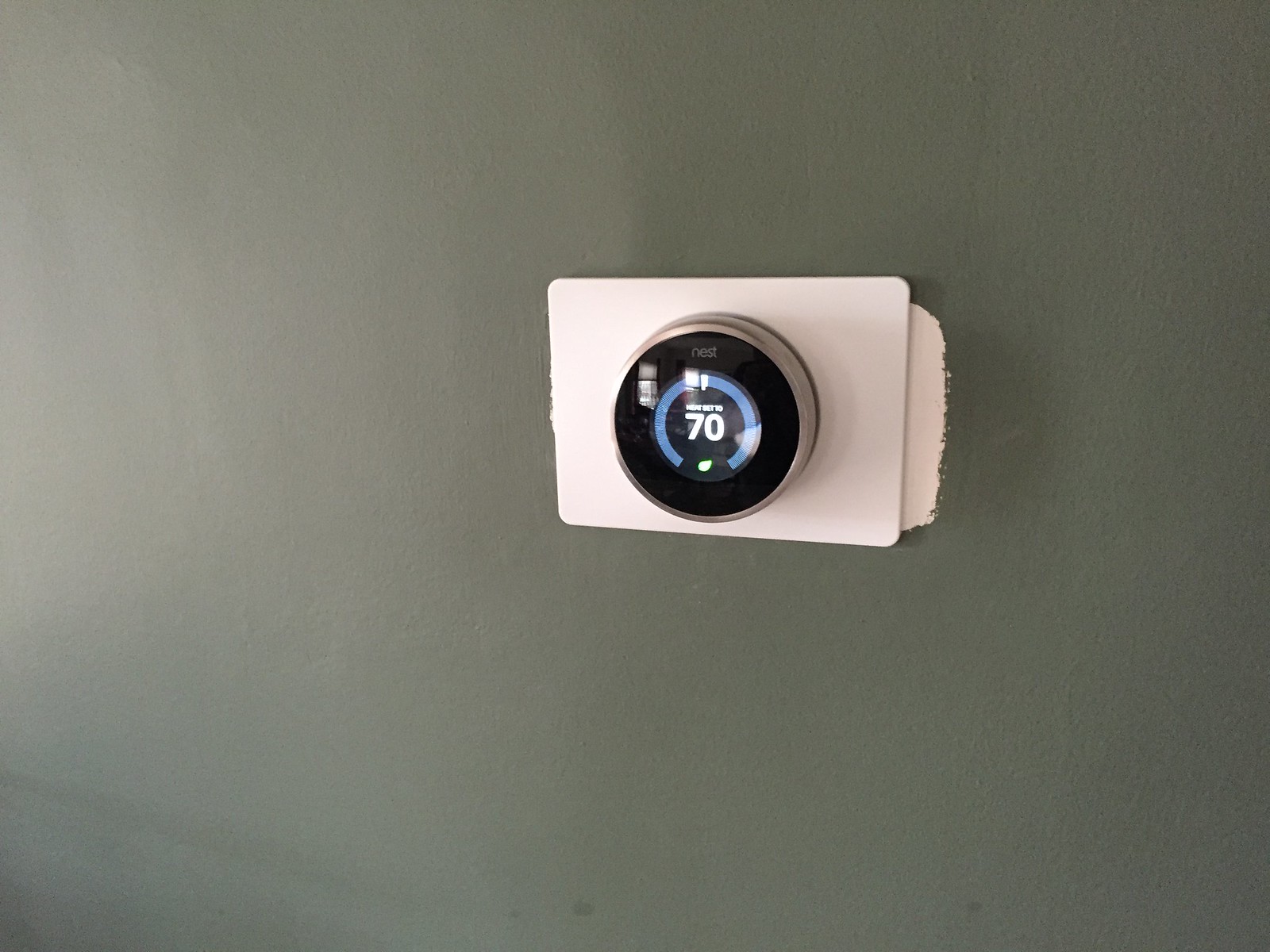The image showcases a Nest digital thermostat, a sophisticated device known for its high quality and advanced technological capabilities. Notably part of Nest’s smart home products line—including items like doorbells—this thermostat can be connected to a smartphone, allowing users to adjust their home's temperature remotely. The device itself is circular, approximately the size of an outstretched palm, featuring a sleek design with a stainless steel outer ring and a black faceplate. 

The display shows a clear, blue line, potentially indicative of the current mode or status, somewhat akin to life meters in video games. A prominent "70" is displayed, likely representing the set temperature. The minimalistic design lacks visible buttons or dials, suggesting that it is primarily controlled via touch or an app.

The installation appears quite recent, as evidenced by the exposed area around the device where the older, smaller fixture’s presence is still marked by edging in the gray paint on the wall, contrasting with the previous white paint underneath. The surrounding wall, painted in a modern gray hue, enhances the sleek aesthetic of the newly installed Nest thermostat.